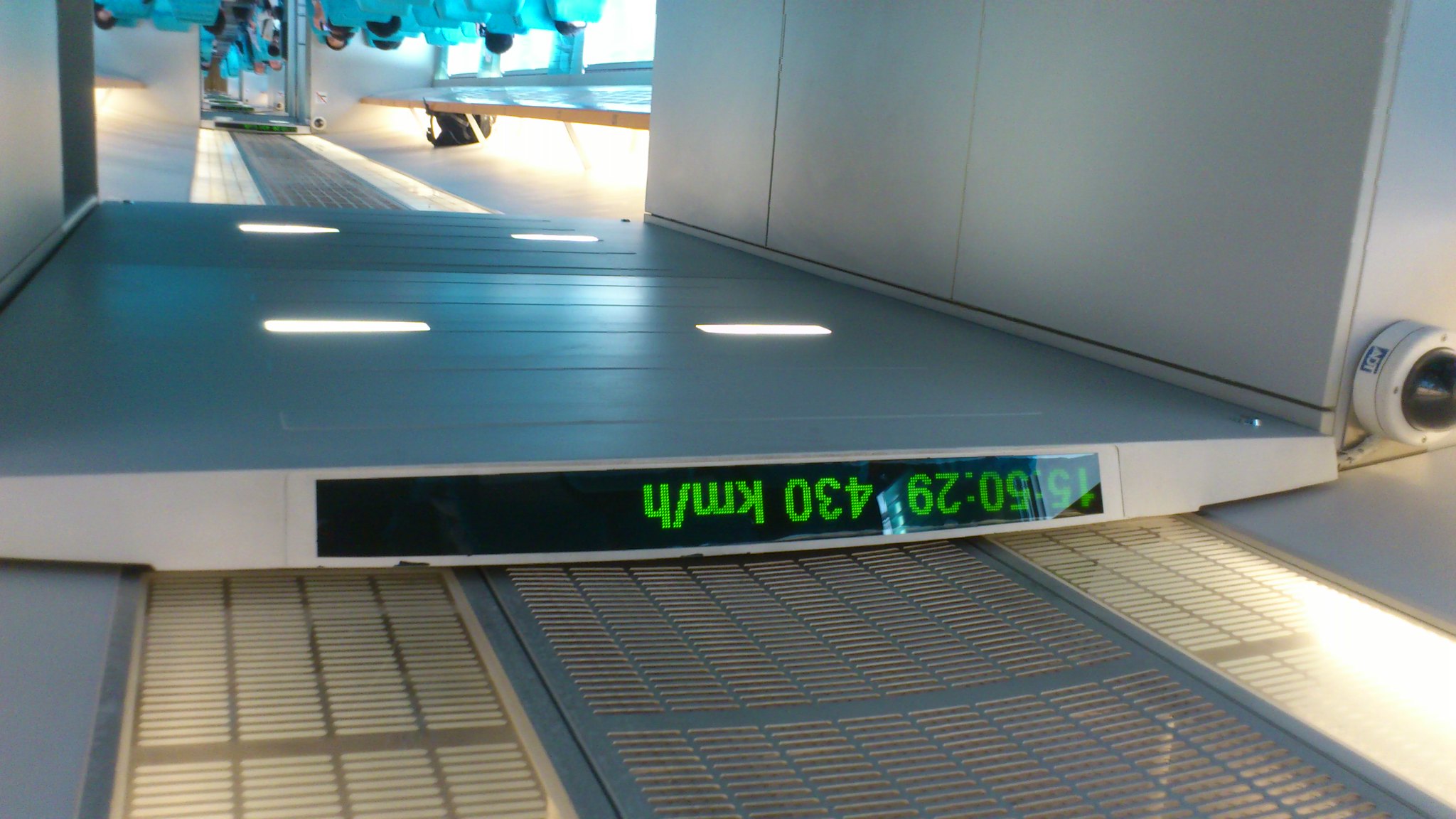The image depicts an inverted perspective, likely showing a passageway that leads to an airplane, with floor and ceiling positions swapped. The focal point is a timestamp reading "15:50:29" and a speed indicator of "430 km/h," both illuminated in green light. Inside the tunnel-like structure, the interior of an airplane is visible, populated by people and what appear to be flight attendants dressed in light blue uniforms. Adjacent to the time display, there is a device resembling a camera, contributing to the array of visual details in the scene.